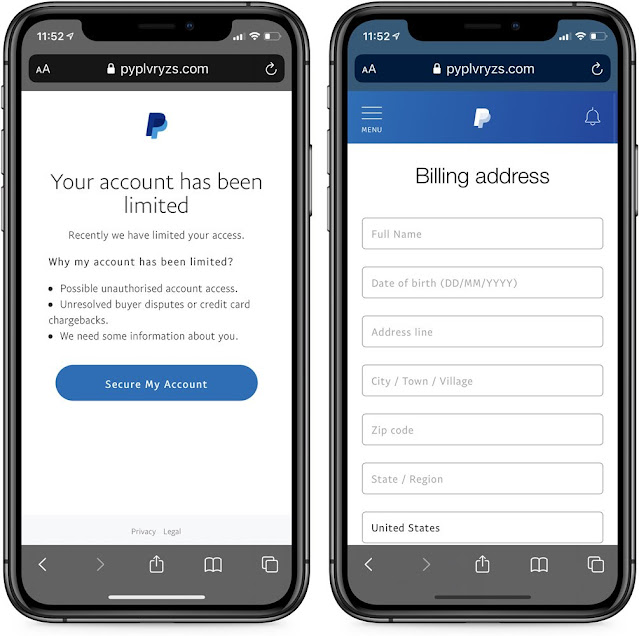The image displays two cell phones placed side by side, both showing the same web address at the top of the screens: pypl.vryzs.com. The time displayed on both phones is 11:52, with the battery level at approximately 30% and four bars indicating signal strength.

In the first phone's screenshot:
- The background is dark gray.
- At the top left corner, the time is shown in white text as 11:52.
- The top right corner displays the battery level (approx. 30%) and signal strength (four bars).
- Below the status bar, there is a black address bar featuring a closed padlock icon, indicating a secure connection, followed by the web address: pypl.vryzs.com.
- Beneath the address bar is a vertical white rectangular box containing the PayPal logo at the top.
- Below the logo, in black text, it says "Your account has been limited."
- Further down, in smaller blue text, it reads, "Recently we have limited your access."
- Following this, in bold navy text, there is a question, "Why My Account Has Been Limited?"
- Three bullet points in blue text outline possible reasons:
  1. Possible unauthorized account access
  2. Unresolved buyer disputes or credit card chargebacks
  3. We need some information about you
- At the bottom, there is a bright blue button with the text "Secure My Account" in white.

In the second phone's screenshot:
- The layout is similar, showing the same web address and time.
- The background is bright blue, displaying the PayPal logo.
- Below the logo, there is a white box containing the label "Billing Address" in black text.
- Underneath, several white boxes outlined in light gray are stacked vertically for input fields:
  1. Full Name
  2. Date of Birth
  3. Address Line
  4. City/Town/Village
  5. Zip Code
  6. State/Region 
  7. At the bottom, there is a box labeled "United States."

This detailed depiction suggests the image may illustrate a phishing attempt designed to mimic PayPal's user interface, aiming to collect personal information from unsuspecting users.